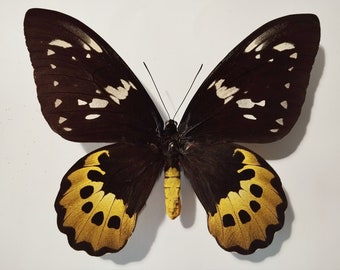This is a top-down view of a beautiful butterfly set against a light gray, solid-colored background, casting a drop shadow down and to the right. The butterfly’s body is predominantly black at the top, transitioning to yellow towards the tail. Its symmetrical wings feature intricate details: the larger top wings are black with splashes of white and small clusters of white dots near the center and edges. The smaller bottom wings are black, bordered by a rippled black edge, and adorned with golden yellow ends that showcase half-oval shapes and four distinct black spots within the yellow area. Thin, black antennae extend from the butterfly's head, completing its delicate appearance.